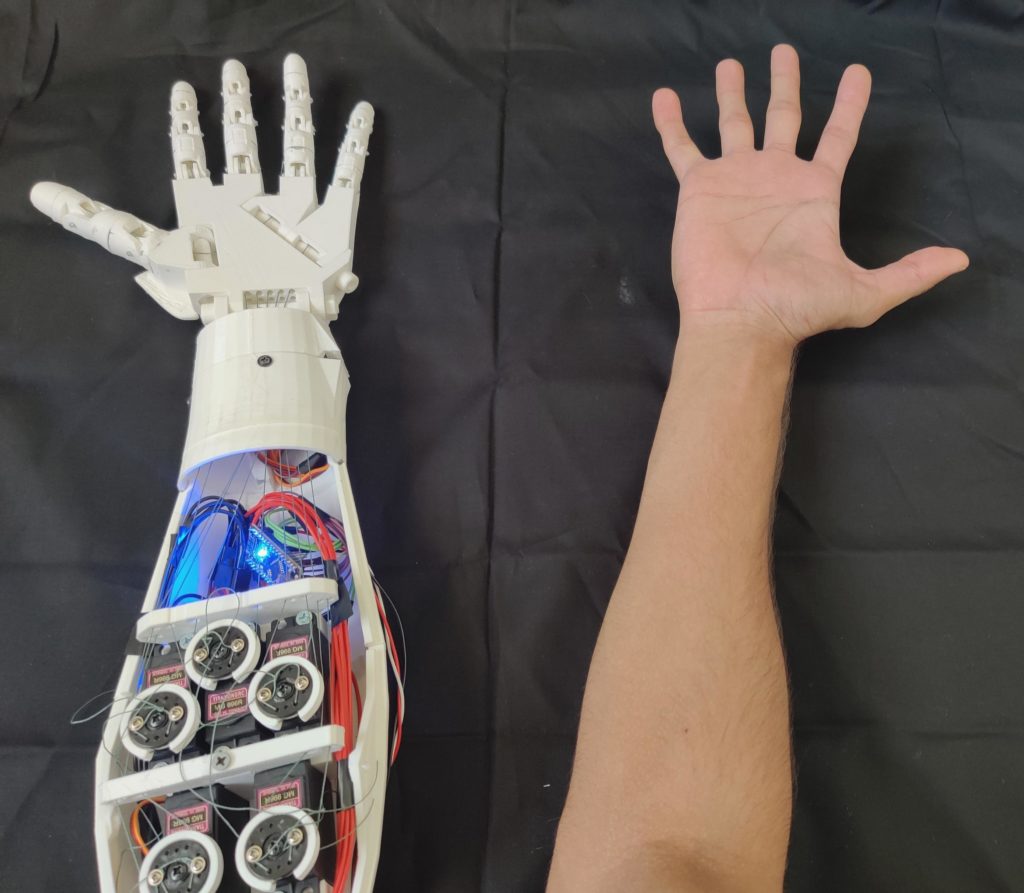The photograph captures a striking juxtaposition of a human arm and a robotic arm, both positioned side by side on a dark fabric surface. The image spans from the elbows to the tips of the fingers, with both hands oriented palm-up and their fingers splayed out. The human arm, located on the right, displays a palm with visible creases and slightly pale skin tone. In contrast, the robotic arm on the left is constructed from white plastic, showcasing intricate details such as joints and a reinforced plastic wrist cap.

The mechanical arm's palm features various divots, adding texture to its otherwise smooth exterior. Moving upwards from the wrist, half of the robotic limb is exposed to reveal its inner mechanisms: an array of wires covered in blue and red plastic, small metal components, batteries, and a glowing blue LED light. Each segment of the arm is meticulously separated by plastic dividers and secured with screws and connectors, illustrating a sophisticated design that emphasizes both its functional and aesthetic aspects. This detailed depiction highlights the convergence of human anatomy and advanced robotics, presenting a compelling comparison of organic and artificial limbs.